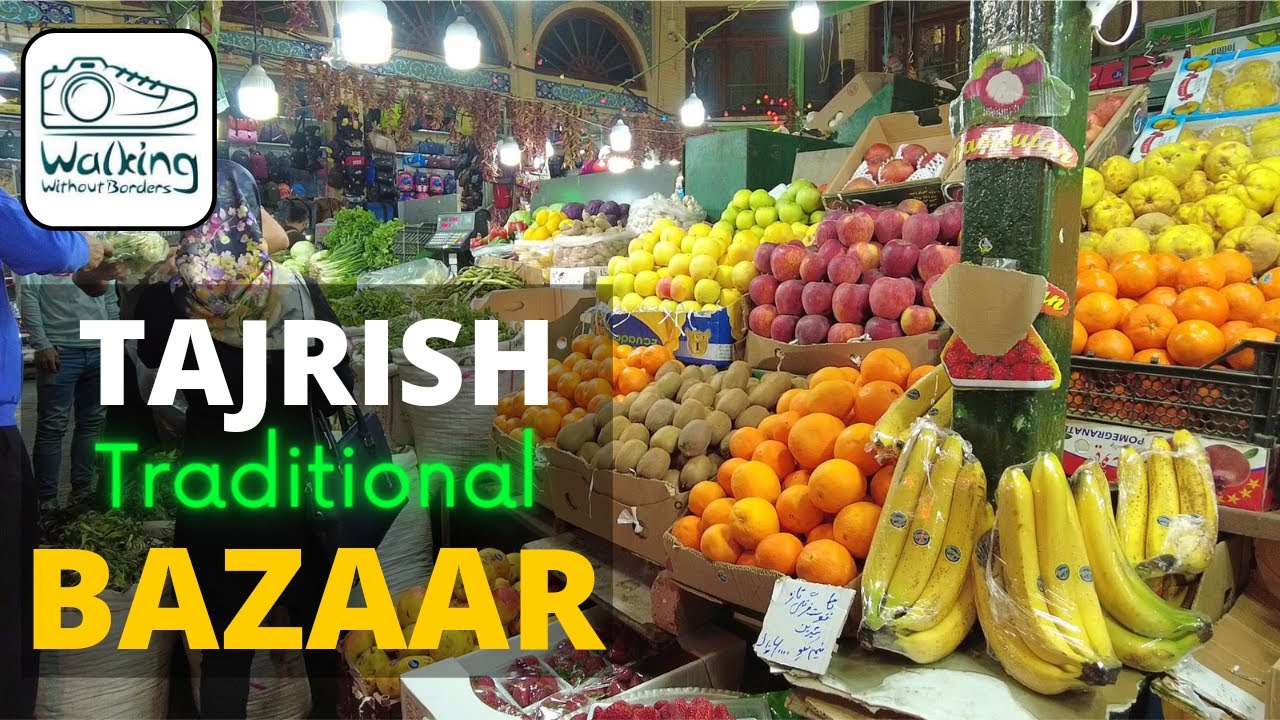The image depicts the bustling interior of the Tajrish Traditional Bazaar. In the foreground, a prominent sign reads "Tajrish Traditional Bazaar," situated just below an inset image in the top left-hand corner that displays the logo "Walking Without Borders" on a white background. The scene is warmly lit, highlighting the intricate pillars and archways that frame the numerous market stalls.

To the right in the foreground, a vibrant display of fresh fruit takes center stage; plump oranges, crisp apples, curved bananas, and fuzzy kiwis are neatly arranged. Smaller fruits, such as ripe raspberries and strawberries, are also visible, adding further splashes of color. On the left side, an array of vegetables is organized in contrasting shades of green and other earthy tones. The background reveals additional stalls, each piled high with an abundance of goods, emphasizing the market's rich and varied offerings. The ambient lighting and the energetic atmosphere capture the inviting allure of this traditional marketplace.